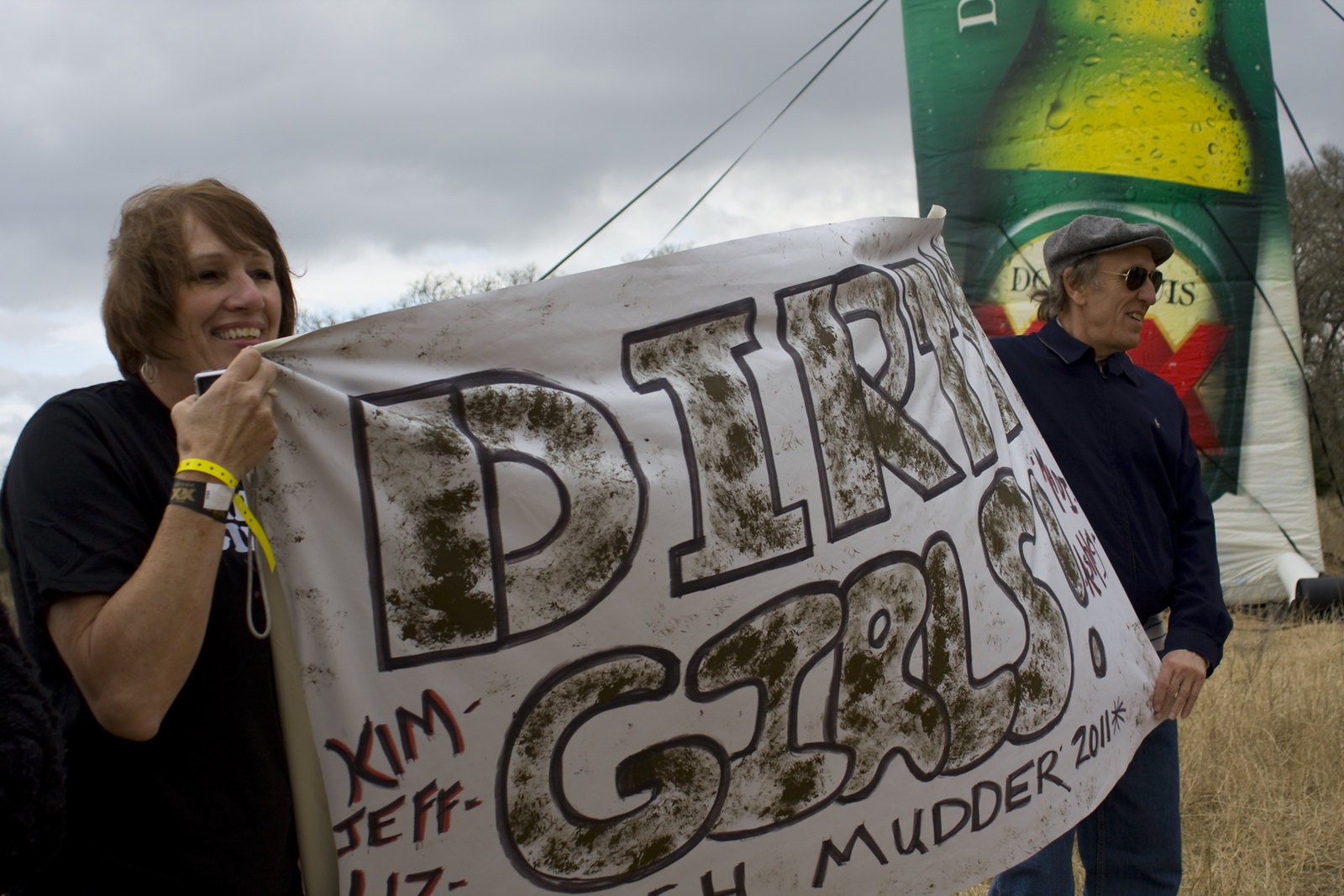In this vibrant outdoor daytime scene, a smiling woman and a man are proudly holding a homemade, hand-printed banner at an event called "Mudder" in 2011. The large, white cloth banner, adorned with text that looks like it’s smeared with mud and dirt, reads "Dirty Girls Mudder, 2011." Various names like Kim, Jeff, and Liz are scrawled along the edges of the banner, though some names are partially cut off. The woman, standing to the right, is dressed in a black shirt and sports various colorful bracelets and a yellow wristband, indicating event participation. She has short brown hair. The man, on the left, is dressed in a dark top and jeans, and accessorized with sunglasses and a gray flat cap. Behind them looms a colossal inflatable Dos Equis beer bottle, complete with guy wires for stability, and vivid condensation details that evoke a refreshing allure. The entire scene is set against a backdrop of grassy terrain and clear skies, capturing a moment of enthusiasm and camaraderie.